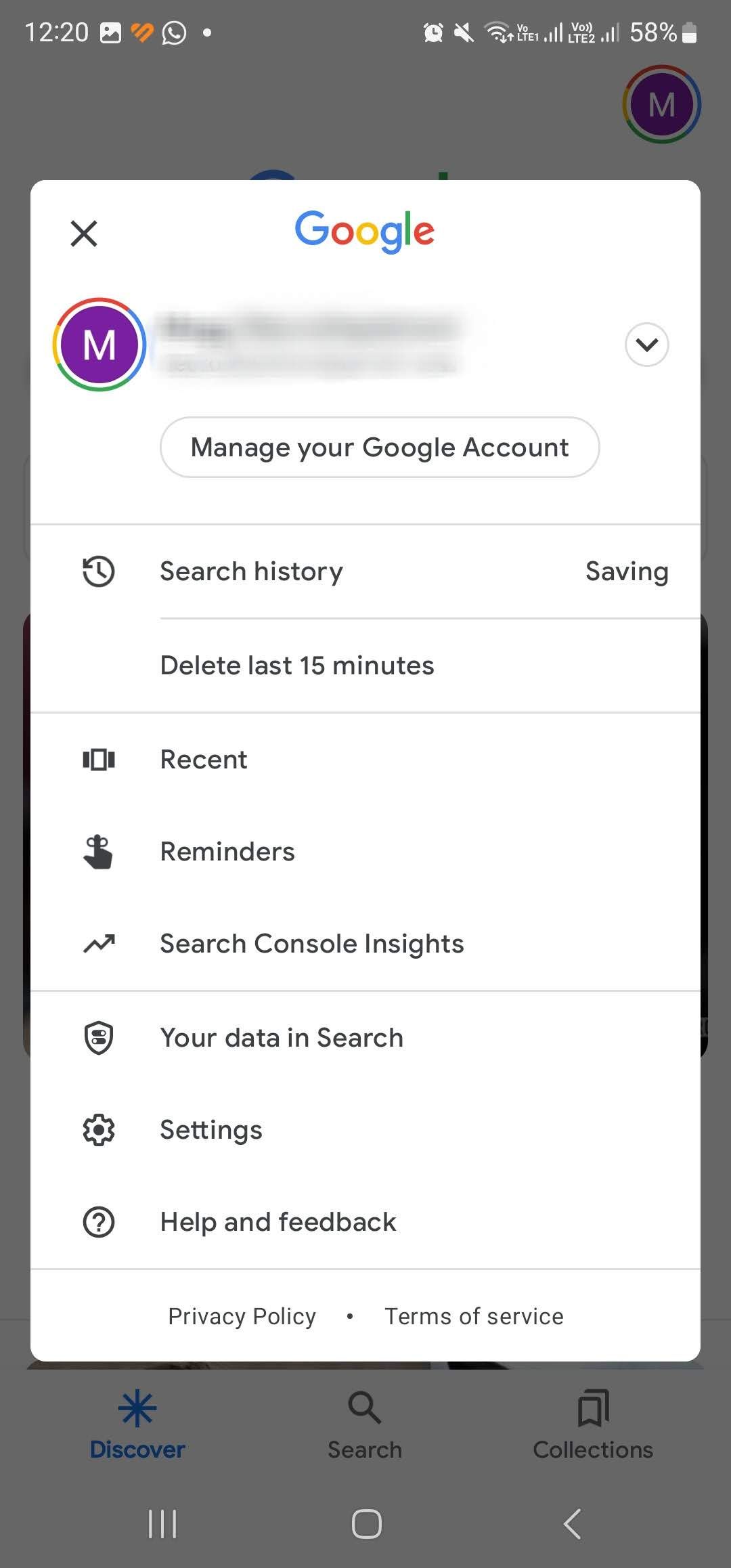The background of the box is predominantly gray. At the upper right corner, there is a purple circle containing the letter "M". Just above this circle, the battery life is displayed at 58%. On the top left, the time is shown as 12:20. Next to the time, there's a long white oval with an "X" in its upper left corner and the word "Google" beside it.

Directly beneath this, there is a repeat of the letter "M" inside a purple circle, followed by the text "Manage your Google Account." Below this line, there's an icon of a clock inside a circle next to the words "Search history and saving." Continuing down, you'll find the option "Delete last 15 minutes."

Further down, the options listed are: "Recent," "Reminders," "Search Console Insights," and "Your data in Search." Accompanying these text options is a gear icon labeled "Settings" and a question mark inside a circle titled "Help and feedback."

At the very bottom, transitioning back to the gray background, there are three options: "Discover" in blue on the left, a magnifying glass icon with the word "Search" underneath in the center, and a set of 3D-styled squares with the word "Collections" below it on the right.